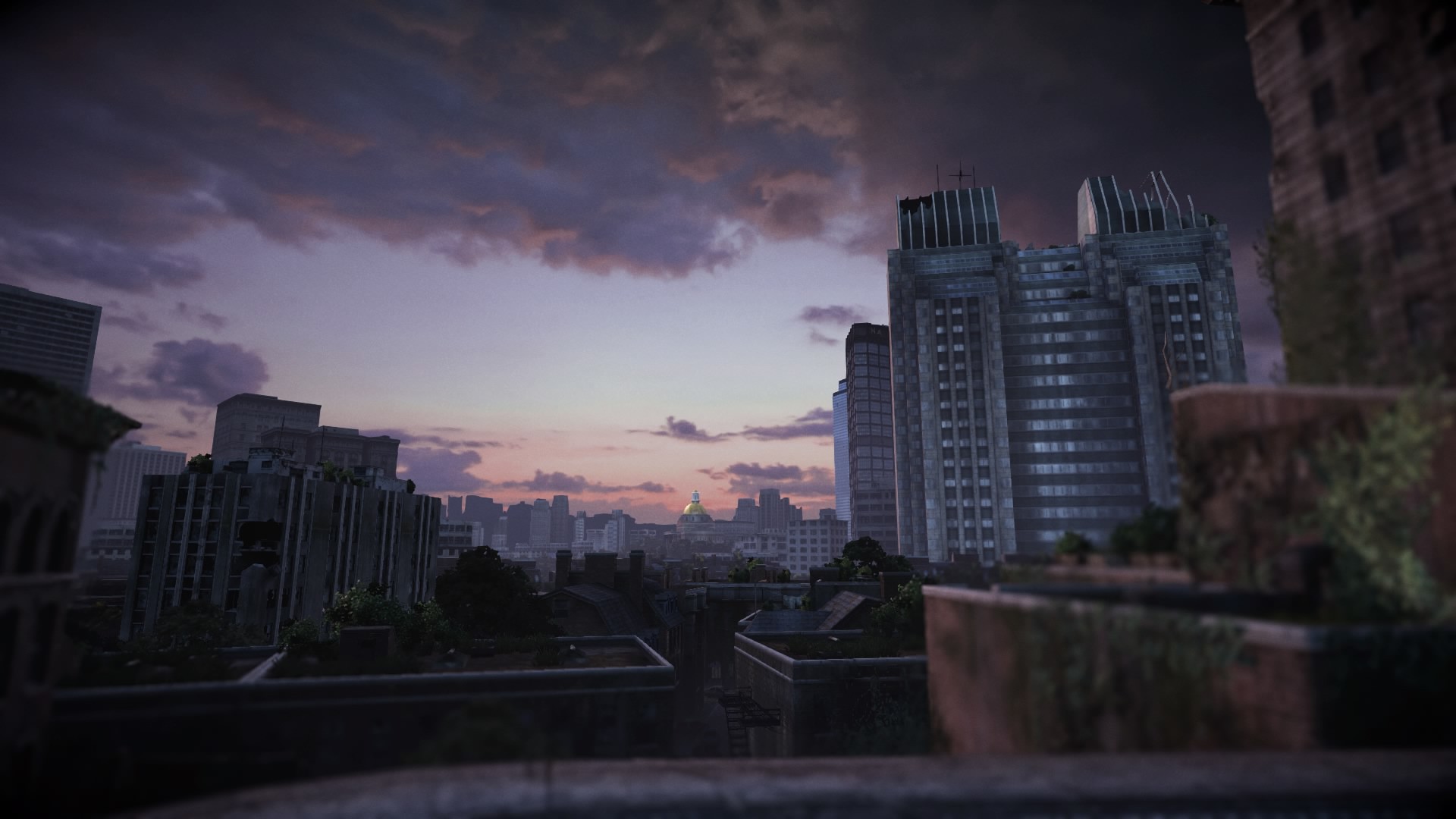This AI-generated image presents a cityscape at dusk or dawn, bathed in a pinkish-orange, dusky lavender sky with scattered, multi-hued clouds in shades of purple and mauve. The horizon showcases a serene pink color. The city itself has an abandoned, forlorn feel, accentuated by the visible damage on several buildings concentrated on the left side. In the foreground, there are rooftop gardens with trees, though somewhat blurred, hinting at a greening effort. 

Dominating the background is a golden-domed building that resembles a capital with a spire, surrounded by other tall structures. A prominent gray building with shiny windows and distinct top panels stands out. Another shorter building is positioned behind it, while additional tall buildings, possibly apartments, feature what appear to be sheds or air conditioning units on their rooftops. From the viewpoint, a reddish concrete flower planter suggests the photo is taken from a balcony, adding to the intricate urban depth of the scene.